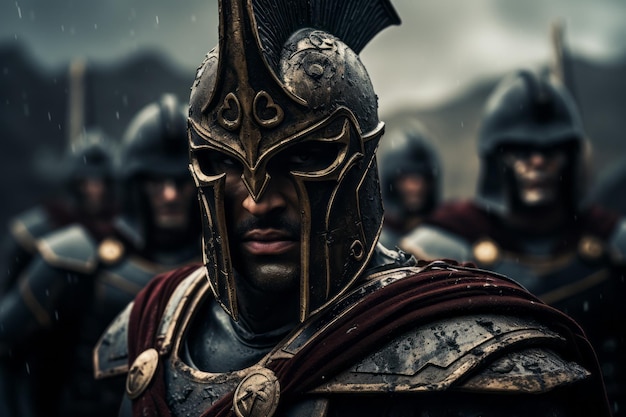The image is a detailed, artistic representation of a soldier, reminiscent of Spartan or Greek warriors. The central figure is a dark-skinned man with intense, determined eyes, suggesting readiness for battle. He is adorned in armor that is a dark metallic gray trimmed with gold, evoking the appearance of bronze or brass. His helmet is particularly striking, wrapping around the entire face except for cutouts around the eyes down to the mouth and nose, and it features a distinctive mohawk-like crest. His shoulders are protected by metal shoulder plates, and two medallions anchor a blood-red fabric that drapes over his shoulders and forms a cape. 

In the blurred background, there are other soldiers wearing simpler, open-faced black helmets with minimal design, and their armor is predominantly black with gold edges. The setting appears to be outdoors during the daytime, possibly in inclement weather such as snow or rain, with indistinct hills in the distance. The overall scene conveys a sense of an ancient, formidable army prepared for battle, with the foreground soldier commanding focus with his fierce, intent expression.